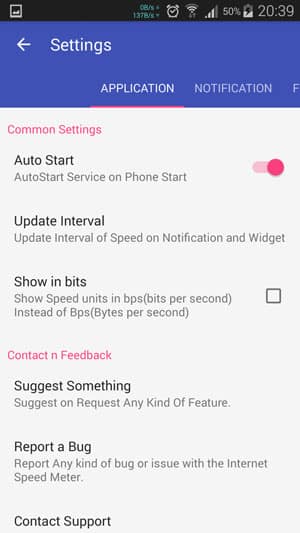This is a screenshot taken from a smartphone displaying a settings menu. At the top of the screenshot is a half-inch black border. In the top-left corner, a white outline of a square with a black inside is visible. To the right of this icon, the time "20:39" is displayed in white. Next to the time, a half-full battery icon with a charging symbol indicates 50% battery life. Adjacent to the battery icon are four full Wi-Fi signal bars. There's also an alarm clock icon and, beside it in blue text, "CB/S" with "137B/S" beneath it. 

Below this top bar, there is a two-inch section of dark blue background. In the left corner of this section, a white left-pointing arrow is situated next to the word "Settings" in large white letters. Directly below "Settings," the word "Application" is displayed in white, and to the right of it, "Notification" is partially visible, with the letter "F" extending off the right side of the screen. A red line appears under "Application."

The remaining part of the screenshot transitions to a light gray background. In the top-left corner of this gray section, the text "Common Settings" is displayed in red. Below, "Auto Start" is written in bold black, followed by the phrase "Service on Phone Start" in regular black text. To the right of this line, a red toggle switch is shown in the "on" position.

Moving down the left side, "Update Interval" is written in bold black letters, and the text "Update Interval of Speed on Notification and Widget" is displayed in regular black text beneath it. Further down, "Bits" appears in bold black letters next to a black-bordered square. Below, "Contact and Feedback" is written in red. "Suggest Something" follows in bold black text, and underneath it, a regular black line describes the suggestion feature. The words "Report a Bug" are also bolded in black, with two regular lines detailing the report procedure beneath it. At the very bottom, the text "Contact Support" in bold black is partially visible, trailing off the bottom of the screenshot.